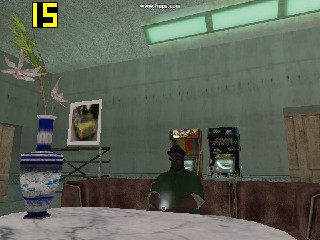The scene is set in a video game environment characterized by a predominantly gray backdrop, including gray walls and a ceiling. Large windows with a greenish tint occupy part of the wall, casting a subtle hue across the room. In the upper left corner, a yellow number "15" is prominently displayed. From the ceiling, various objects are suspended, adding to the room's complexity. Adorning the wall is a picture frame, while below, a sizable table with a marbled white and gray surface is surrounded by brown chairs. Seated at the table is an individual wearing a black hat, accompanied by video arcade machines—a brown one and a black one—positioned behind them. The walls also feature light brown curtains, contributing to the room's ambiance.